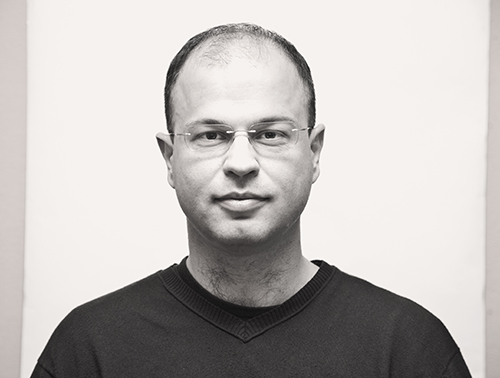This black-and-white photograph captures a close-up of a middle-aged man from the chest up, centered in the frame against a white background with two vertical gray strips on either side. The man, who appears to be in his 40s, has a balding head with a thin layer of very short brown hair that recedes from the top to the sides, with a few strands adorning his forehead. His face is adorned with small wire-rimmed glasses, showcasing his brown eyes that gaze directly at the camera. He has a wide nose, a slight smile with closed lips, and a dimple in his chin. A smattering of hair extends up from the front of his neck. He is dressed in a dark V-neck t-shirt, which seems to have some stitching issues on the left side. The overall composition gives a stark yet intimate portrayal of the subject, emphasizing the contrast and details within the monochromatic palette.